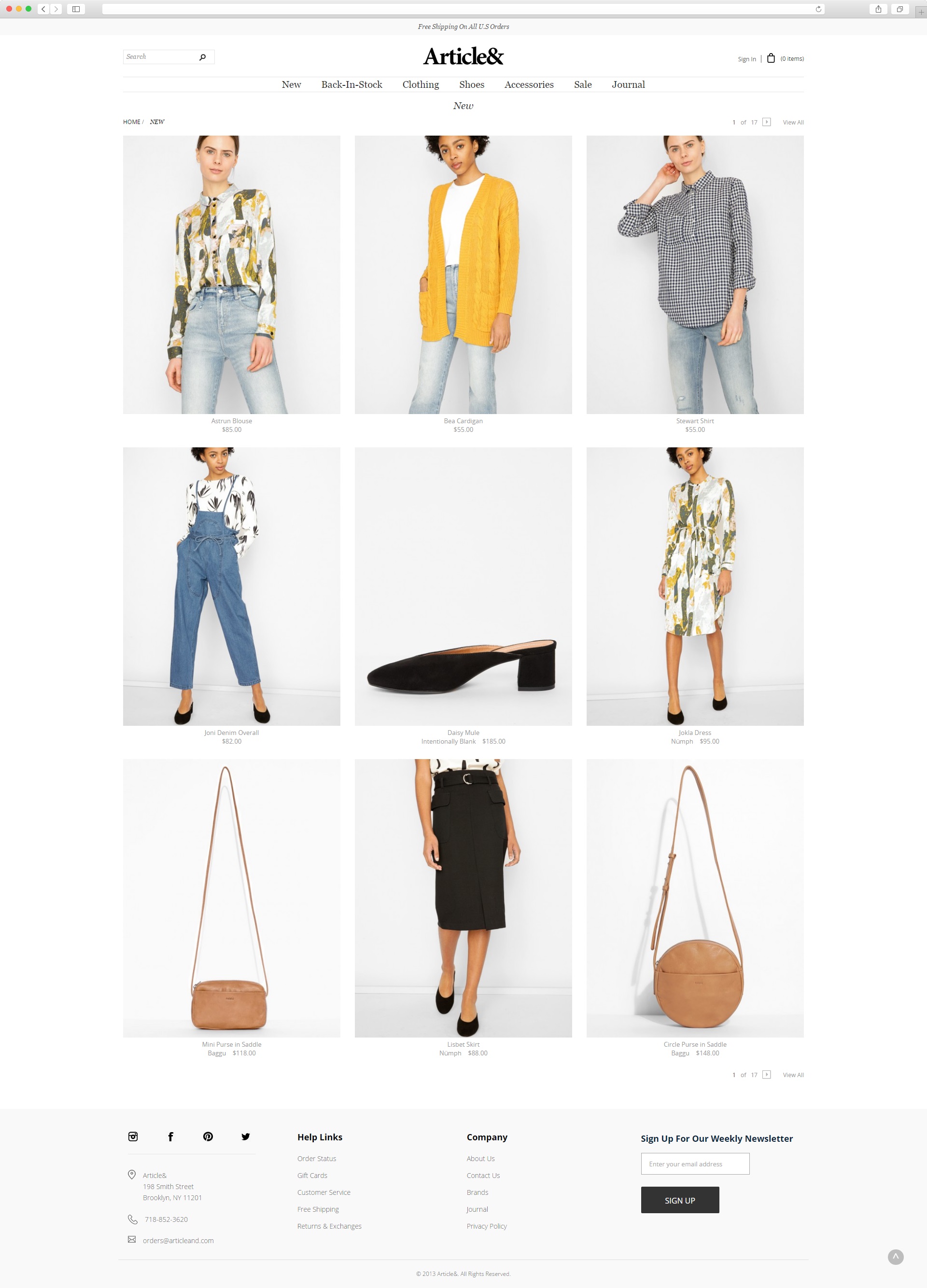The webpage appears to be from an online clothing store. The header section of the page is white, featuring the store's name, "Article &," centered in black text. Beneath the header, there is a navigation menu offering options such as "Back in Stock," "Clothing," "Accessories," "Shoes," and "Sale."

The main section of the page displays a grid of nine rectangular images. In the upper left, there's an image of a woman wearing light blue jeans paired with a long-sleeve shirt featuring gray and yellow hues. Moving to the right, the next image shows another woman in light blue jeans and a yellow sweater. The third image in the top row also features a woman in light blue jeans, this time paired with a black-and-white button-up shirt.

In the second row, starting from the left, there is an image of a woman dressed in blue overalls and a white shirt adorned with a plant pattern. The central image showcases a black high-heeled shoe, and to its right is a woman wearing a white long-sleeve dress with green and yellow accents.

The bottom row features a pink, rectangular-shaped purse, followed by an image of a black skirt, and concluding with a circular pink purse.

At the bottom of the page, which has a gray background, there are links to the store's social media handles and various help options.